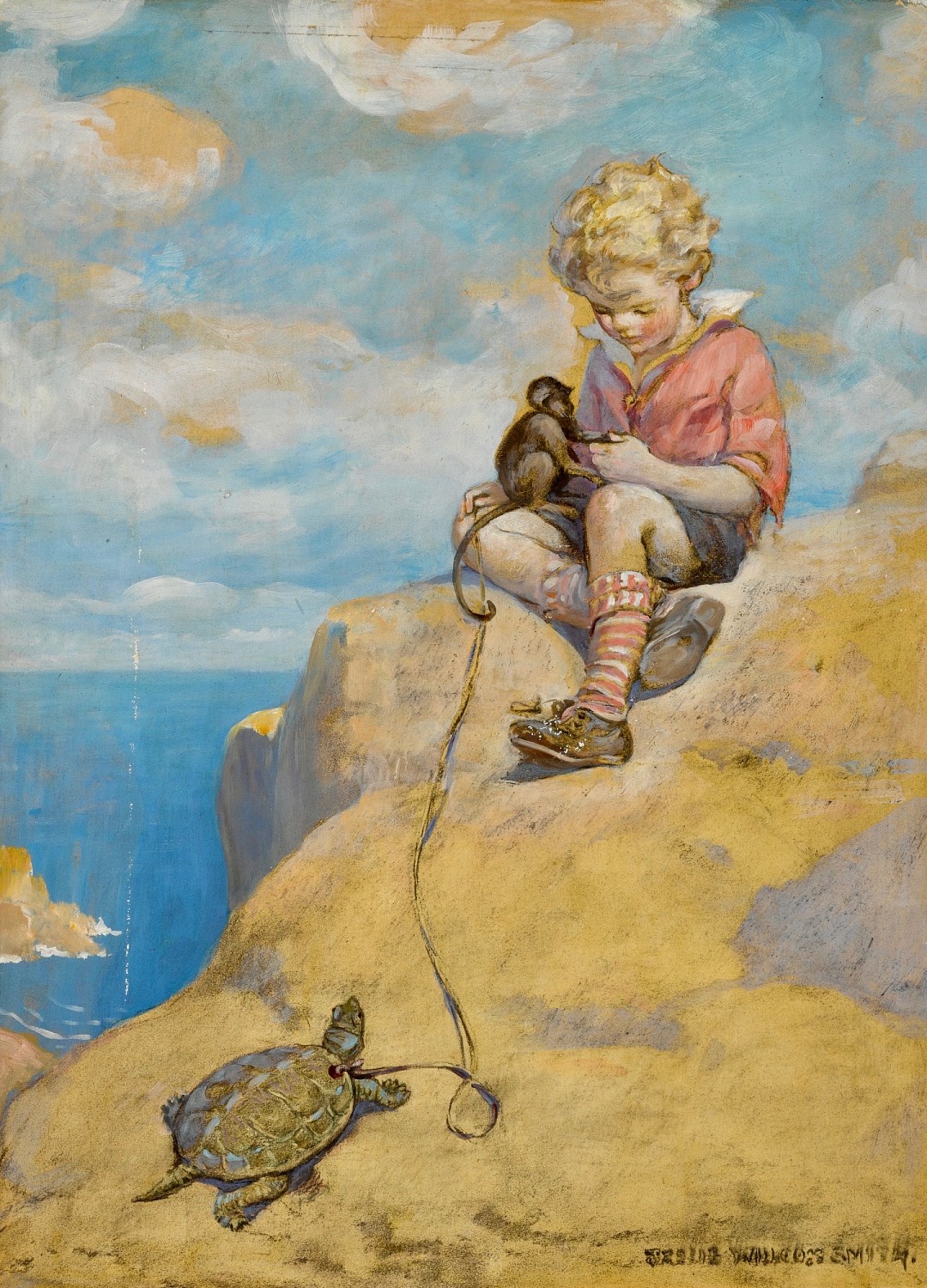In this detailed painting, a small blonde child, possibly a young boy, is seated on a large, light brown rock that overlooks a deep blue body of water on the left. The child is wearing a distinctive outfit consisting of blue shorts, knee-high striped red and white socks, brown shoes, and a red sailor-type shirt with a white collar. Sitting on the child's lap, particularly his right leg which is crossed under his left leg, is a small monkey. The child is holding a string that is tied directly to the shell of a turtle, which is walking towards him from further down the rock. The background features a sky of billowy blue and white clouds with hints of yellow. The painting includes an artist's signature in the bottom right corner, with the last name "Smith" clearly visible, while the first and middle names are indistinct.